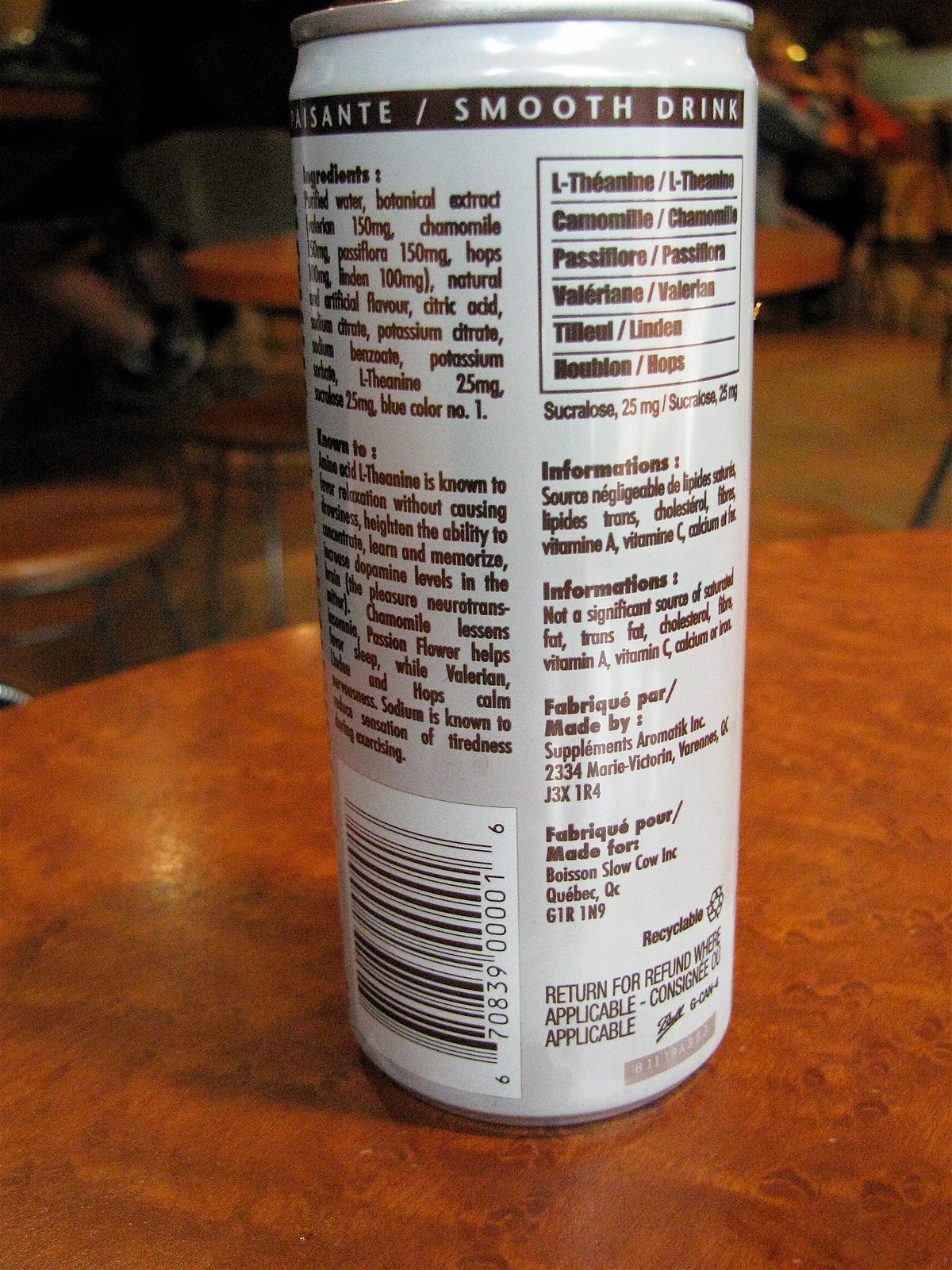In this rectangular image, we see a close-up of a narrow, round can positioned on a dark brown wooden table or countertop. The can is predominantly white with a silver top and we are viewing the back side, which features the nutritional label. The barcode situated in the lower left corner is printed in dark brown against the white background.

Along the top of the label, the product is identified as "Smooth Drink." The listed ingredients include water, botanical extract, chamomile, potassium, citric acid, and artificial flavoring. There's also a note mentioning the presence of the amino acid theanine, which is known for promoting relaxation without causing drowsiness, enhancing concentration, learning, memorization, and increasing dopamine levels. The description goes on to highlight the benefits of other ingredients: chamomile for soothing effects, passionflower for aiding sleep, and valerian and hops for calming nervousness.

The label also includes product and company details. The section in the lower right corner states, "Fabrique Pour / Made for Boisson Slow Cow Inc., Quebec G1R 1NN." Additionally, the can is marked as recyclable.